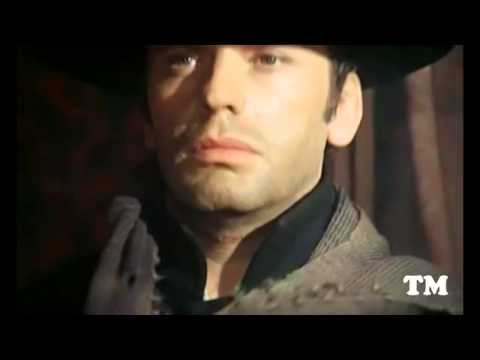This is a full-color photograph set against a solid black background, bordered by thicker black margins on the top and bottom, and thinner ones on the sides. The image features a close-up of an adult Caucasian male's head and shoulders. He has dark brown hair, brown eyes, and long sideburns with a 5 o'clock shadow, giving a faint hint of stubble. The man's skin is slightly tan, and he appears to be in his 30s, with an intense look of concentration on his face as he gazes off to the right side of the camera, lips closed and no particular expression.

He is wearing a black high-collared shirt with rounded collars, possibly of a vintage or ornate style, and over it, a grayish-purple jacket that hints of intricate detailing, possibly with lace trim and high shoulders. The top of his head is slightly cut off but reveals he is wearing a black hat, which could be a cowboy or bolero hat. The overall impression of his attire suggests it may be from a classic Western or period film, perhaps evoking themes of the Southwestern border.

On the right side of the image are swirly, brown and tan curtains, lending a dramatic backdrop to the scene. Light illuminates the right side of his face, while the left side is shrouded in shadow, adding depth and intensity to his appearance. The lower right-hand corner of the image contains the only text: the white capital letters "T M." Together, these details create the sense that this might be a still from an old or stylistically vintage film.